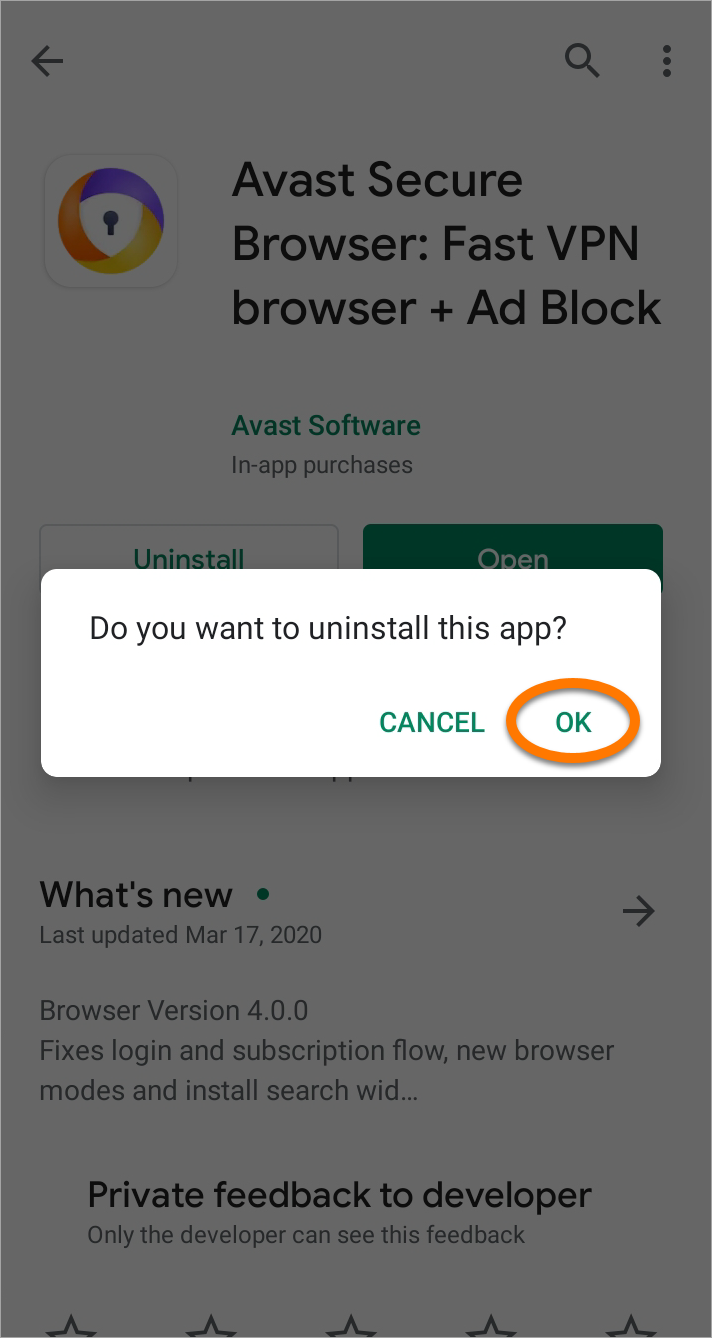The image presented is a vertical screenshot, approximately three times taller than it is wide, captured from a mobile device. The entire background is overlaid with a semi-transparent gray, focusing attention on the primary content in the foreground.

At the top-left corner, there's a black left-pointing arrow icon, while the top-right corner displays a magnifying glass icon next to a vertically arranged trio of dots. Below these icons, a distinct logo featuring three interlocking colors—blue, yellow, and orange—encircles a small key lock symbol. Adjacent to the logo, bold text reads: "Avast Secure Browser: Fast VPN Browser + Ad Block." This indicates the screenshot is taken from a download page for the Avast Secure Browser.

Further down, the text "Avast Software" appears in green, with "In-app purchases" noted in black underneath it. Two buttons, spaced apart, are partially visible below this text. The left button, labeled "Uninstall," is white with green text, suggesting that the app is already installed. The right button is green with white text that says "Open."

Dominating the central area of the image is a white rectangular pop-up dialog box, which slightly obscures the bottom part of the two buttons. This dialog, in black text, prompts: "Do you want to uninstall this app?" To the right of this prompt, two options are presented: "Cancel" and "OK", both written in green. The "OK" option is highlighted by an artificially drawn orange circle, indicating this screenshot might be used as an instructional guide for uninstalling the app from a website.

This detailed scene conveys the essence of a user interface for managing the Avast Secure Browser on a mobile device.